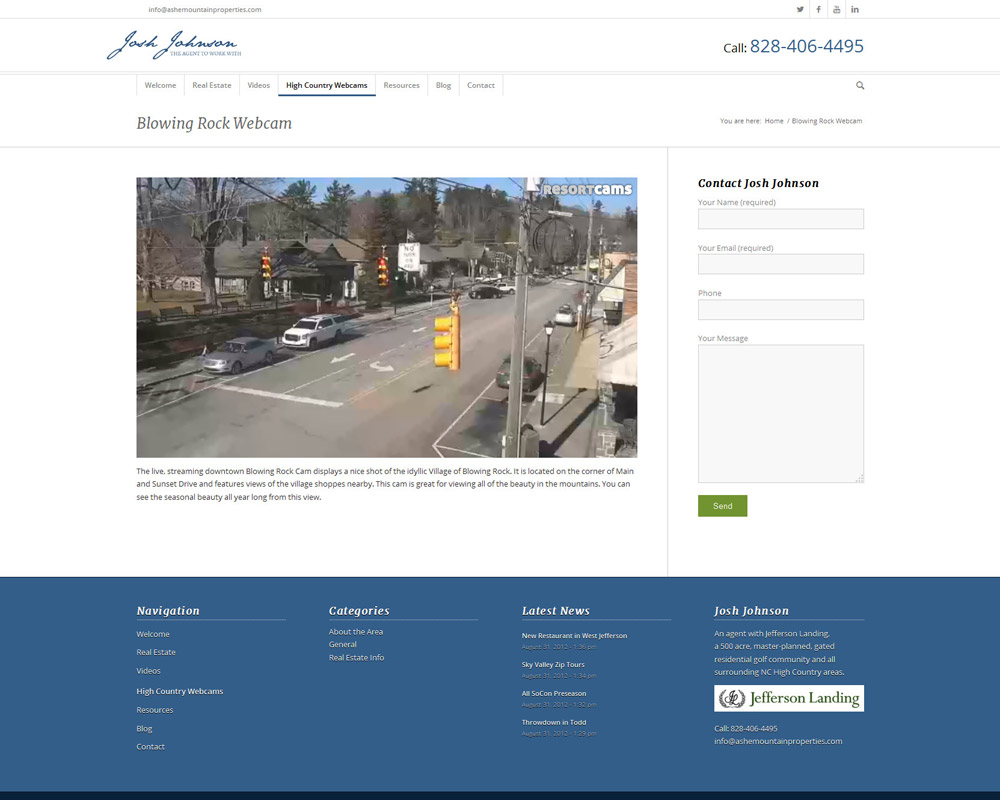The website belongs to Josh Johnson, who appears to work within the realm of real estate. The resolution of the webpage is somewhat lacking, resulting in difficulty reading the text due to its small font size. 

On the right side of the webpage, there's a contact number: 828-406-4495. Above this, social media icons for Twitter, Facebook, and Instagram are displayed. Underneath Josh Johnson's name, the menu options "Welcome," "Real Estate," "Video," "High Country Homes," "Resources," "Blog," and "Contact" are listed, with "High Country Homes" being highlighted in black and underlined in blue, while the remaining options are in gray.

The webpage features a "Blowing Rock Webcam" section with a video labeled "Resort Cams" in the upper right corner. This video shows a live feed of an intersection with traffic signals hanging from wires.

Towards the right side of the webpage, there's a contact form labeled "Contact Josh Johnson." The form includes fields for "Your Name" (required), "Your Email" (required), "Phone," and "Your Message," followed by a green "Send" button.

At the bottom of the webpage, a navigation section is present. The leftmost part, titled "Navigation," includes links for "Welcome," "Real Estate," "Videos," "High Country," "Webcam," "Resources," "Blog," and "Contact." Adjacent to this, the "Categories" section lists "About the Area," "General," and "Real Estate Info."